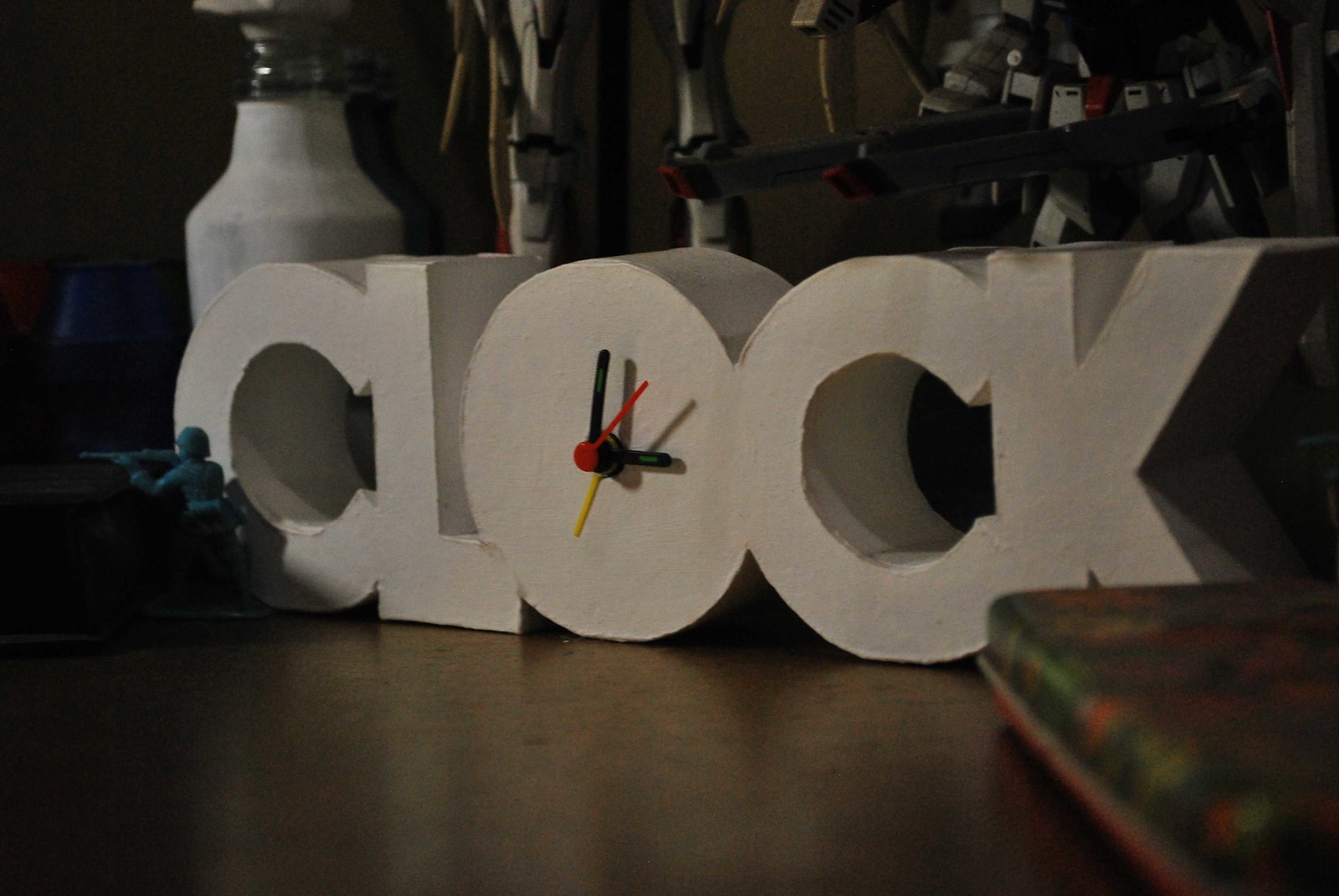The image depicts a brown, reflective countertop with a prominent statue-like clock at its center. The clock, a rectangular block with notable depth, has the word "CLOCK" engraved on it. At the heart of the clock is a cylindrical face showing three hands: the second hand pointing to the top right, the minute hand directed north, and the hour hand positioned in the southeast quadrant. To the bottom right of the clock rests a pillow-like object, while the bottom left houses a small toy-shaped cylinder. In the background, various indistinct objects can be seen, adding a sense of depth and complexity to the scene.